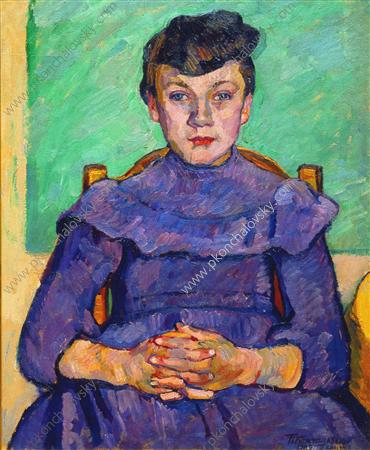The image is a small, vertical rectangular painting of a woman sitting in a wooden chair, facing the viewer. She is depicted from the knees up, with her hands clasped on her lap. The woman is wearing a blue dress with ruffles around the neckline, which extends to her neck, and sleeves that reach past her elbows. The dress features some other colors, possibly purplish tones, and the woman has light skin and dark hair styled up and curled under at the forehead. She wears red lipstick and eye makeup. The chair is brown, and behind her is a green background that resembles a chalkboard, bordered by brown, possibly wooden elements. On the far right of the painting, there is a yellow object near her left elbow, and white diagonal text in the center with the URL www.pkonchalovsky.com. The setting is clear and well-defined, capturing a serene yet striking image of the woman.